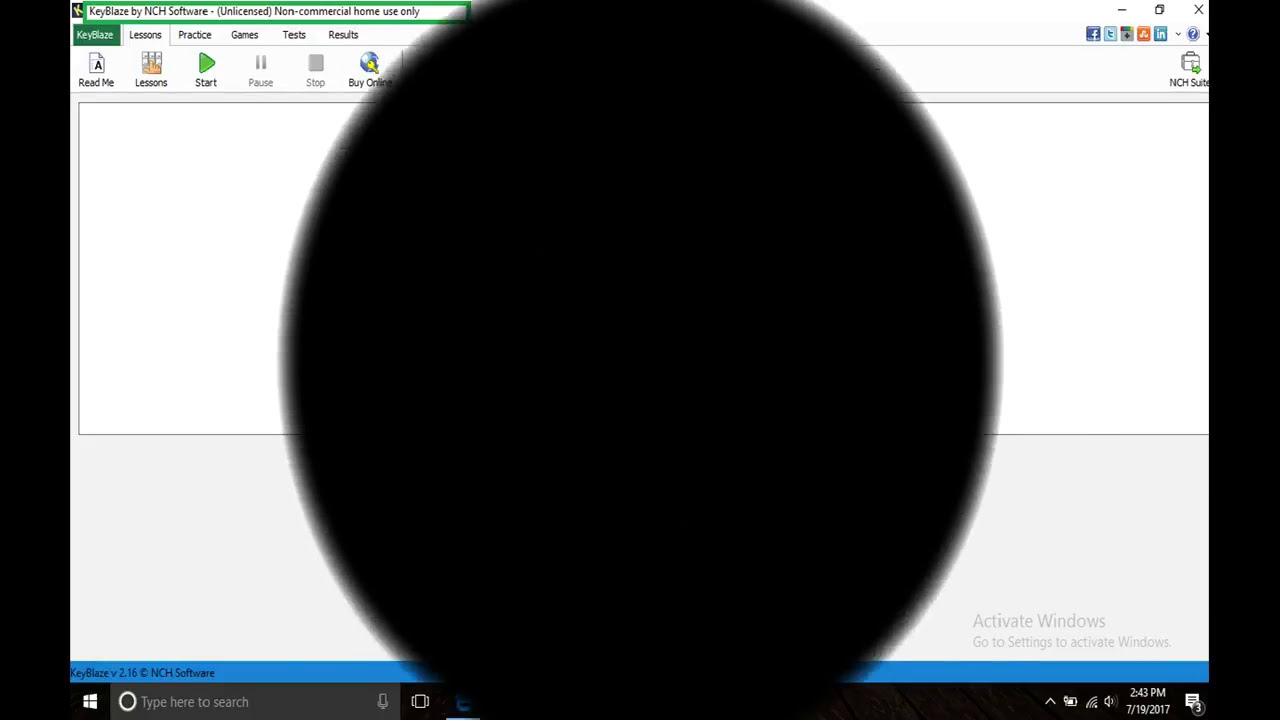This image showcases a snapshot of a Windows computer screen featuring an open program window of Keyblaze by NCH Software, primarily designated for unlicensed non-commercial home use only. The background of the Keyblaze window is predominantly white with gray borders, and it prominently displays a large black circle in the center. The menu options visible on the program include Lessons, Key West, Practice, Games, Tests, and Results. The bottom status bar is marked with a horizontal sky blue line and contains details such as "Keyblaze version 2.16, copyright NCH Software" along with "Microsoft Windows," and it features a search field labeled "type here to search." On the right side of the status bar, there are three notifications, a date and time stamp reading 2:43 PM, July 19, 2017, and a prompt to "activate windows." Additional buttons visible include options like Read Me, Lesson Start, Pause, Stop, or Buy Online.